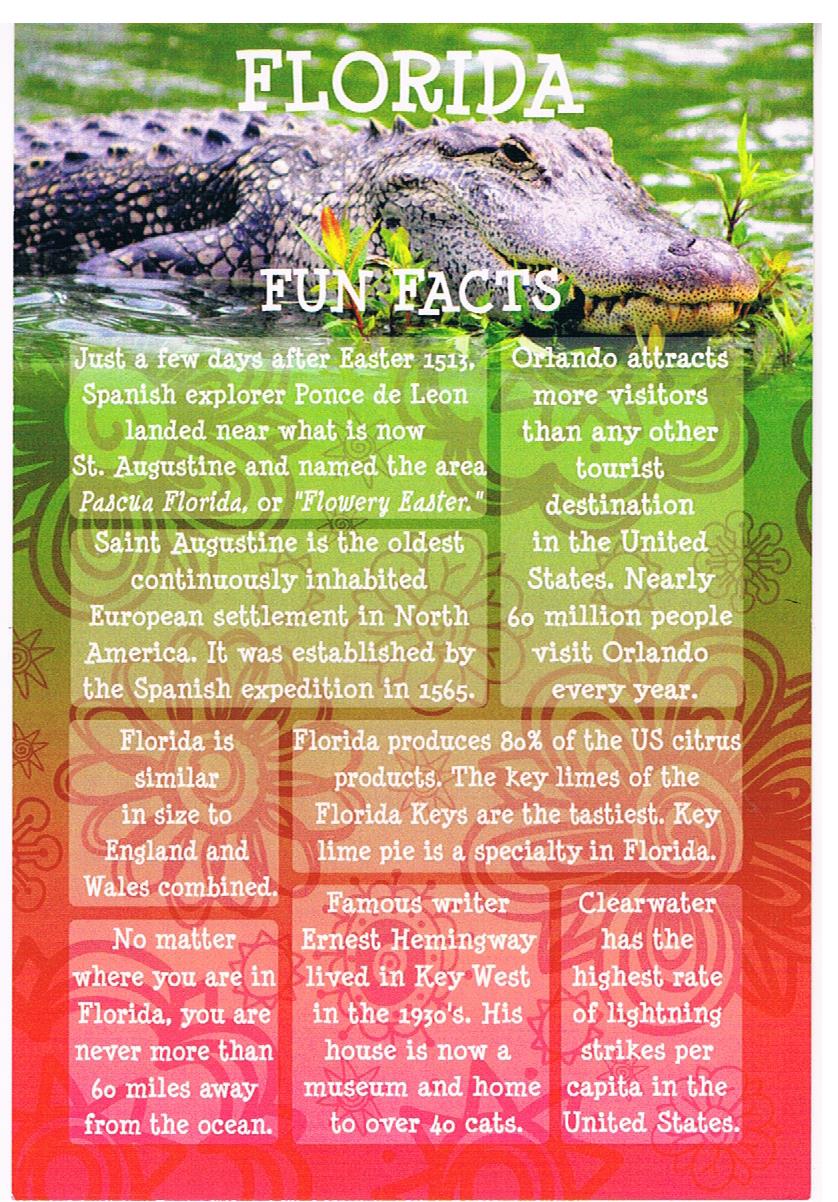The image is a vibrant and detailed advertisement about Florida, crafted in a rectangular layout. Dominating the top of the image is a photograph of an alligator, mostly out of the water, surrounded by green foliage. The word "Florida" sits prominently above the alligator, followed by "Fun Facts" superimposed over the photograph. The background transitions from a green hue at the top, blending into yellowish tones in the middle, and culminating in red, pink, and purple shades at the bottom. This colorful background is adorned with flowery digital designs, adding to the dynamic visual appeal. Below the alligator image are several blocks of white text containing various fun facts about Florida, including historical tidbits such as "Florida is similar in size to England and Wales combined" and notes about St. Augustine being the oldest continuously inhabited European settlement in North America, established by a Spanish expedition in 1565. The informative blocks, about eight in total, are uniformly spaced and provide engaging facts about the state, all set against the ornate and vivid backdrop.